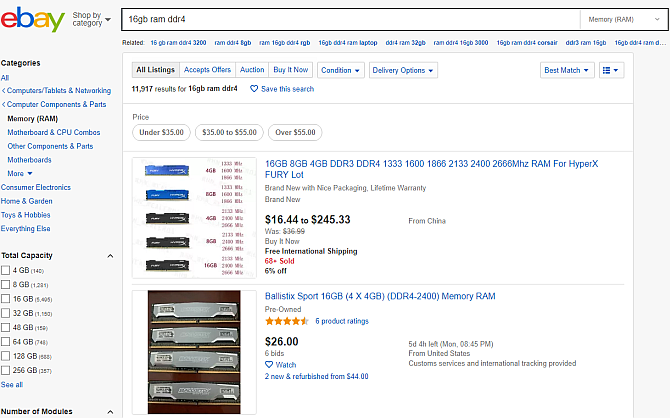A screen capture of an eBay search results page for "16 gigabyte RAM DDR4" is shown. The search query has yielded 11,917 results, indicating a popular item for those looking to upgrade or replace their computer memory. Only two listings are visible in the snapshot, though the webpage continues beyond this capture, suggesting numerous more options. The first listing highlights a lot sale, offering brand new RAM modules with nice packaging and a limited warranty. This seller mentions having five different sizes available, with prices ranging from $16.44 to $245. The second listing features a single 16GB DDR4 RAM module priced at $26.